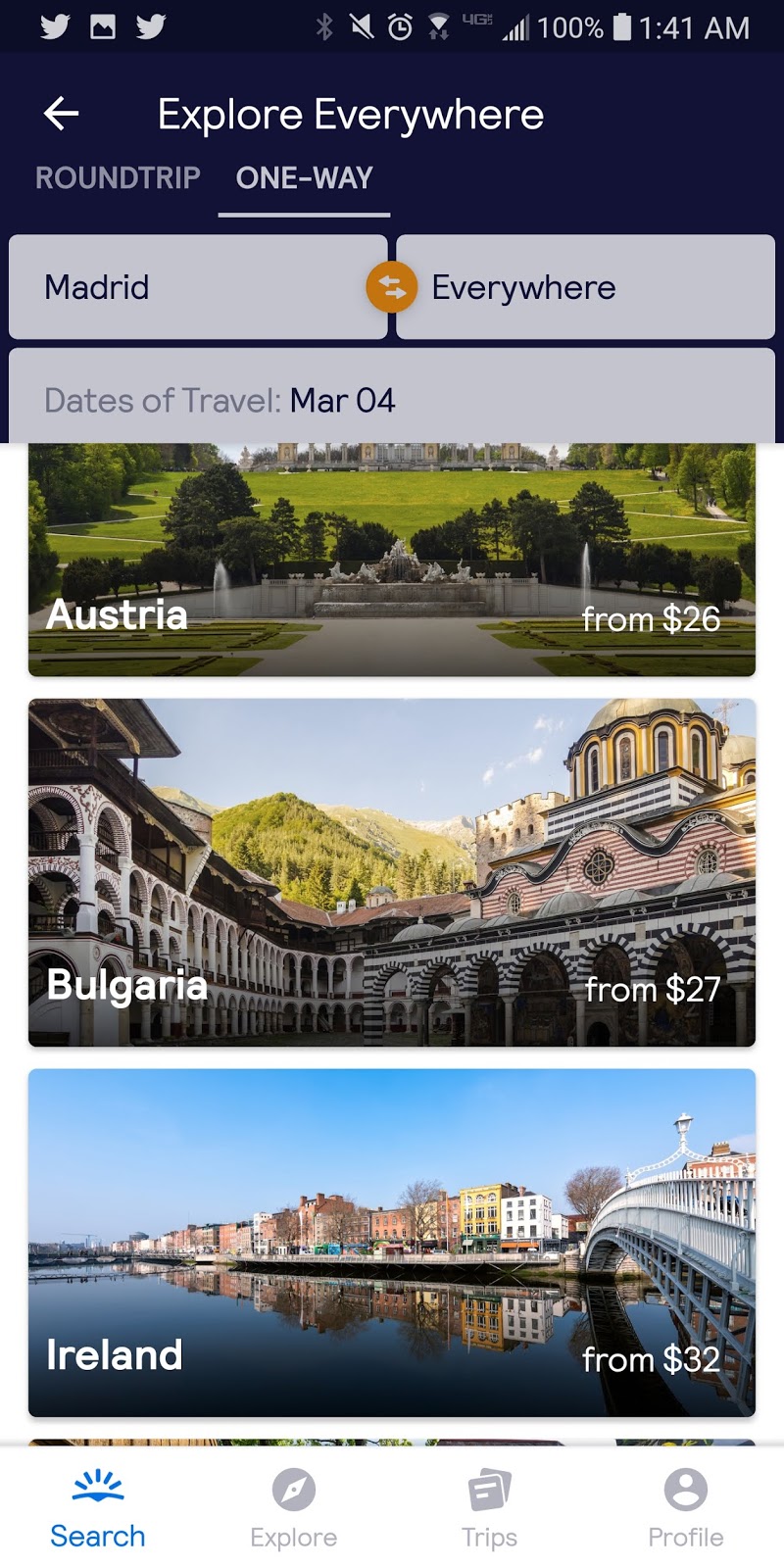This screenshot from a mobile device captures a user navigating the "Explore Everywhere" section of an app, likely related to travel or flight booking. It showcases a rich interface with various icons and options. 

At the top of the screen, the mobile user interface displays a series of icons on a dark blue background, all rendered in white. From left to right, the icons include the Twitter icon, an image icon, another Twitter icon, a space, then Bluetooth, mute, alarm, an unidentified icon, another tiny icon, signal strength showing four out of five bars, the number 100% indicating full battery, a vertical battery icon, and the time stamped at 1:41 AM.

Beneath this, aligned to the left center, the heading "Explore Everywhere" is displayed with a left-pointing arrow, all in white. Just below this, a tab menu is present featuring two options: "Round-tripped" and "One way," with the latter underlined and in a brighter white, indicating its active status.

Directly below the tab menu are two horizontally aligned text fields resembling buttons. The first text field shows "Madrid," and the second texts field, which can be interchanged using a central reverse button, displays "Everywhere." Below these is another field labeled "Dates of travel," populated with "MAR04."

The main content area shows three visible tiles with travel destinations and their starting prices. The first tile features Austria with an image of an elaborate garden, marked with white text "from $26." The second tile shows Bulgaria with text "from $27" and an image of a picturesque scene. The third tile depicts Ireland, showing "from $32" with an accompanying image of a lake by a city and a bridge. A portion of a fourth tile can be seen at the bottom edge.

Finally, the app's navigation bar at the bottom includes four icons: "Search," which is highlighted in blue, indicating its active status, and three grayed-out icons: "Explore" with a compass icon, "Trips" with document icons, and "Profile" with a user icon.